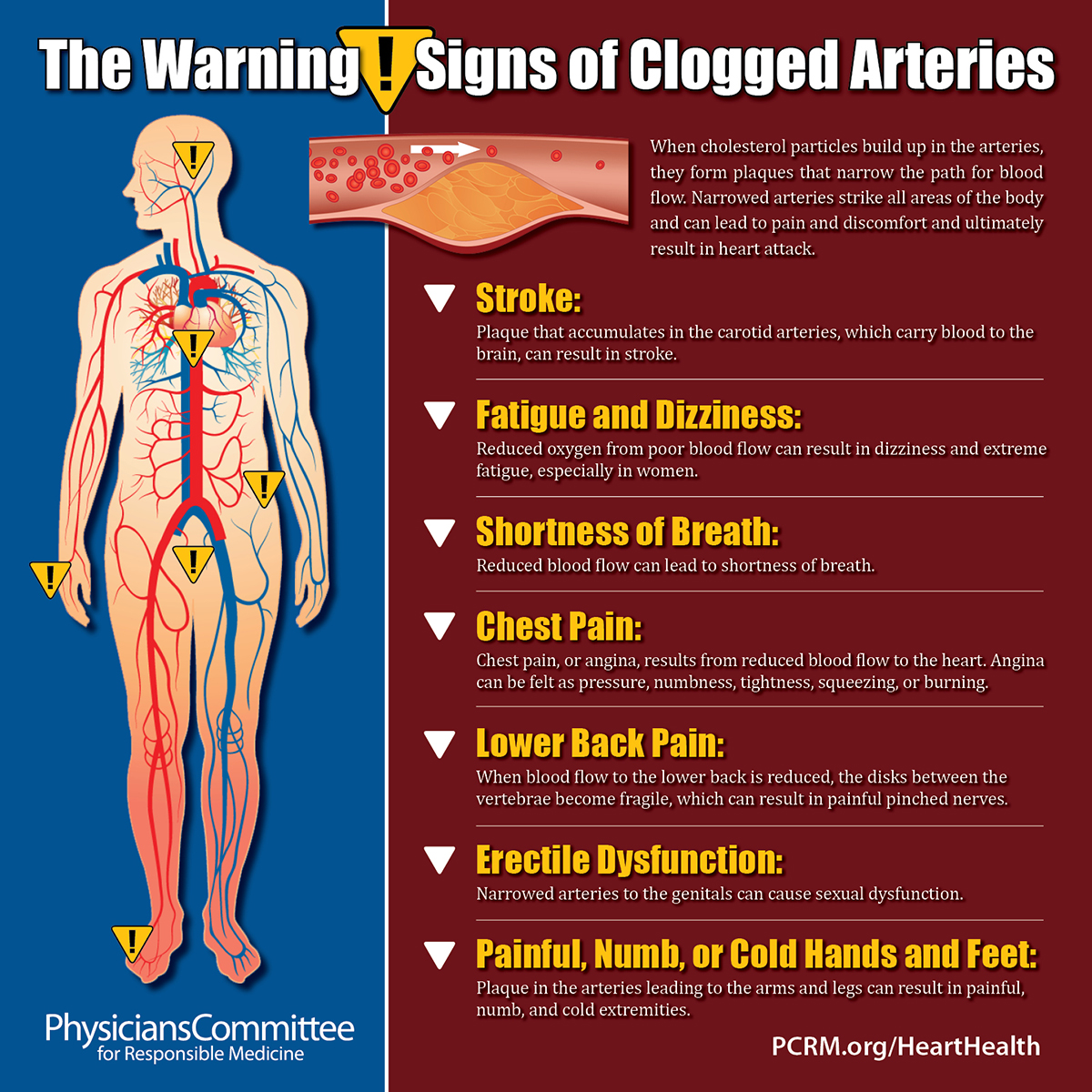This health poster, ideal for display in a doctor's office or pharmacy, is designed to educate viewers on the warning signs of clogged arteries. The layout is split into a blue left column and a dark red right column. The blue section features a detailed human body diagram highlighting the arterial system in red and blue, marked with six yellow warning symbols. Below this diagram, the text reads "Physician's Committee for Responsible Medicine."

The red section of the poster is  labeled at the top with bold white text: "The Warning Signs of Clogged Arteries," accented by a yellow warning sign icon. This section includes an illustrative diagram of a clogged artery alongside an informative paragraph explaining that cholesterol buildup forms plaques, narrowing arteries and potentially leading to serious conditions such as heart attacks.

Further down, the red section lists specific symptoms of clogged arteries, each marked with an upside-down white triangle and bold yellow text. These symptoms are:
- **Stroke**: Plaque in the carotid arteries can reduce blood flow to the brain, increasing stroke risk.
- **Fatigue and Dizziness**: Poor blood flow diminishes oxygen supply, causing dizziness and fatigue, particularly in women.
- **Shortness of Breath**: Narrowed arteries restrict blood flow, leading to breathing difficulties.
- **Chest Pain**: Reduced blood flow to the heart can cause angina, felt as pressure, numbness, tightness, squeezing, or burning.
- **Lower Back Pain**: Insufficient blood flow makes spinal discs fragile, leading to painful pinched nerves.
- **Erectile Dysfunction**: Restricted blood flow to the genitals can result in sexual dysfunction.
- **Painful, Numb, or Cold Hands and Feet**: Poor circulation in the extremities results in pain, numbness, and coldness.

At the bottom of the red section, it provides the URL pcrm.org/hearthealth for further information. This detailed poster aims to raise awareness about the risks and symptoms of clogged arteries, encouraging proactive healthcare.